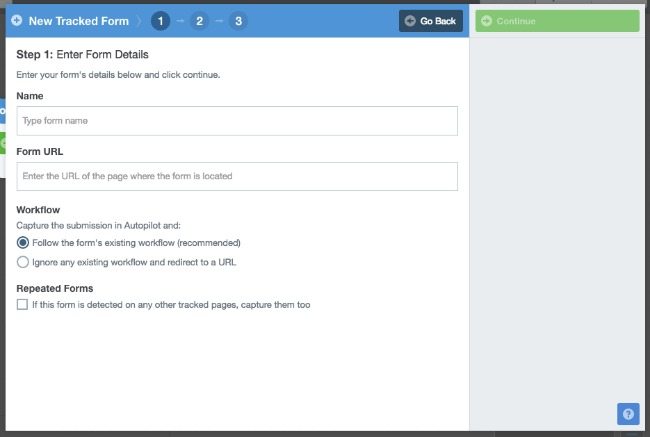This cropped screenshot features a new tracked form box interface. Dominating the top-left corner, a blue bar displays the label "New Tracked Form." Adjacent to this label, there is a small circle with a dark blue plus sign in the center. To the right of "New Tracked Form" is a faint right-pointing arrow leading to a number "1" enclosed in a small blue circle. Subsequent arrows guide to the numbers "2" and "3", each encased in light blue circles.

On the far right, a conspicuous black box contains the text "Go Back." The number "1" is highlighted in a dark blue circle, indicating the current step.

Beneath this highlighted section, the background is white with the heading "Step 1: Enter Form Details" in bold black letters. The instructional text below reads, "Enter your form details below and click continue." Several form fields follow:

- "Name" touted in bold black font, paired with a text box.
- "Form URL" in bold black font, accompanied by another text box.
- "Workflow" in bold black font, followed by the description "Capture the submission in Autopilot" in small black text.

Adjacent to these fields are two side-by-side options:
1. "Follow the form's existing window (recommended)," which is selected.
2. "Ignore any existing window and redirect to a URL," which is not selected.

At the bottom of this section, "Repeated Forms" is emphasized in bold black letters above a checkbox. The text next to the checkbox, "If this form is detected on any other tracked pages, capture them too," remains unselected.

To the right, a gray vertical panel spans the page with a green bar at the top. This bar contains the word "Continue" in small white letters beside a white circle with a green right-pointing arrow. The main body of the page beneath these elements is blank.